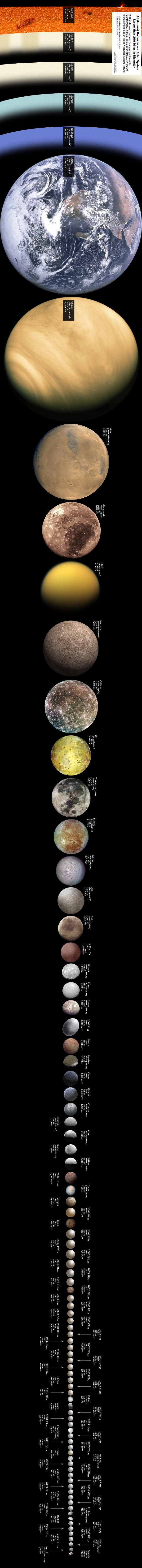The illustration is a tall, rectangular infographic with a black background that showcases Earth's size in relation to all known bodies in our solar system larger than 200 miles in diameter. At the top, a color spectrum including hues like orange, white, light sage, and blue is displayed above the representation of Earth. The planets are depicted in a staggered and vertically stacked alignment, each progressively smaller than the one above, starting with Earth. The diagram continues with the planets transitioning into moons and other celestial bodies as they decrease in size towards the bottom. Alongside the planets, there are Chinese characters and black labels providing additional details. The overall style is a detailed scientific illustration aimed at demonstrating the proportional scale of Earth, other planets, and various moons within our solar system.